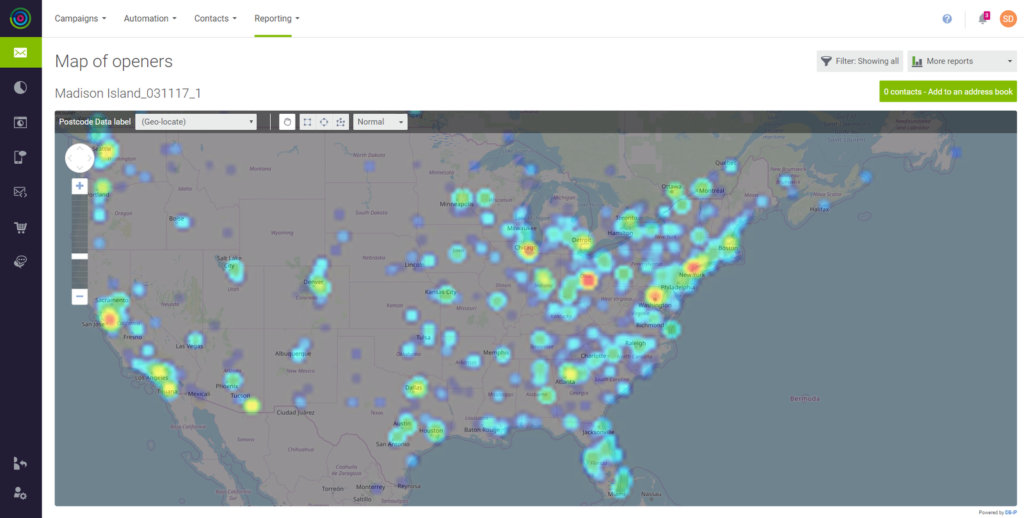The user interface screenshot features a clean, organized design with a predominantly white background at the top area. Displaying key sections titled "Campaign," "Automation," "Contact," and "Reporting." 

On the left side, there is a dark blue vertical menu bar featuring various icons including a moon and a shopping cart, arranged in an up-and-down fashion. Adjacent to this menu, the interface displays a header reading "Map of Openers, Madison Island, _0311117_1."

Positioned below the header, the main visual element is a detailed map of the United States, sprinkled with multiple hotspots located in various regions indicating data points of interest. 

Located at the top right of the interface, there is a bar that includes filter options and another indistinct box with a drop-down menu. Below this, a large green box with unreadable text is visible, suggesting it might contain important metrics or information. 

In the very top-right corner of the interface, a few small, unidentified icons are present, further adding to the interface’s functionality. The overall layout is sleek and purpose-driven, aimed at providing quick access to essential tools and data.